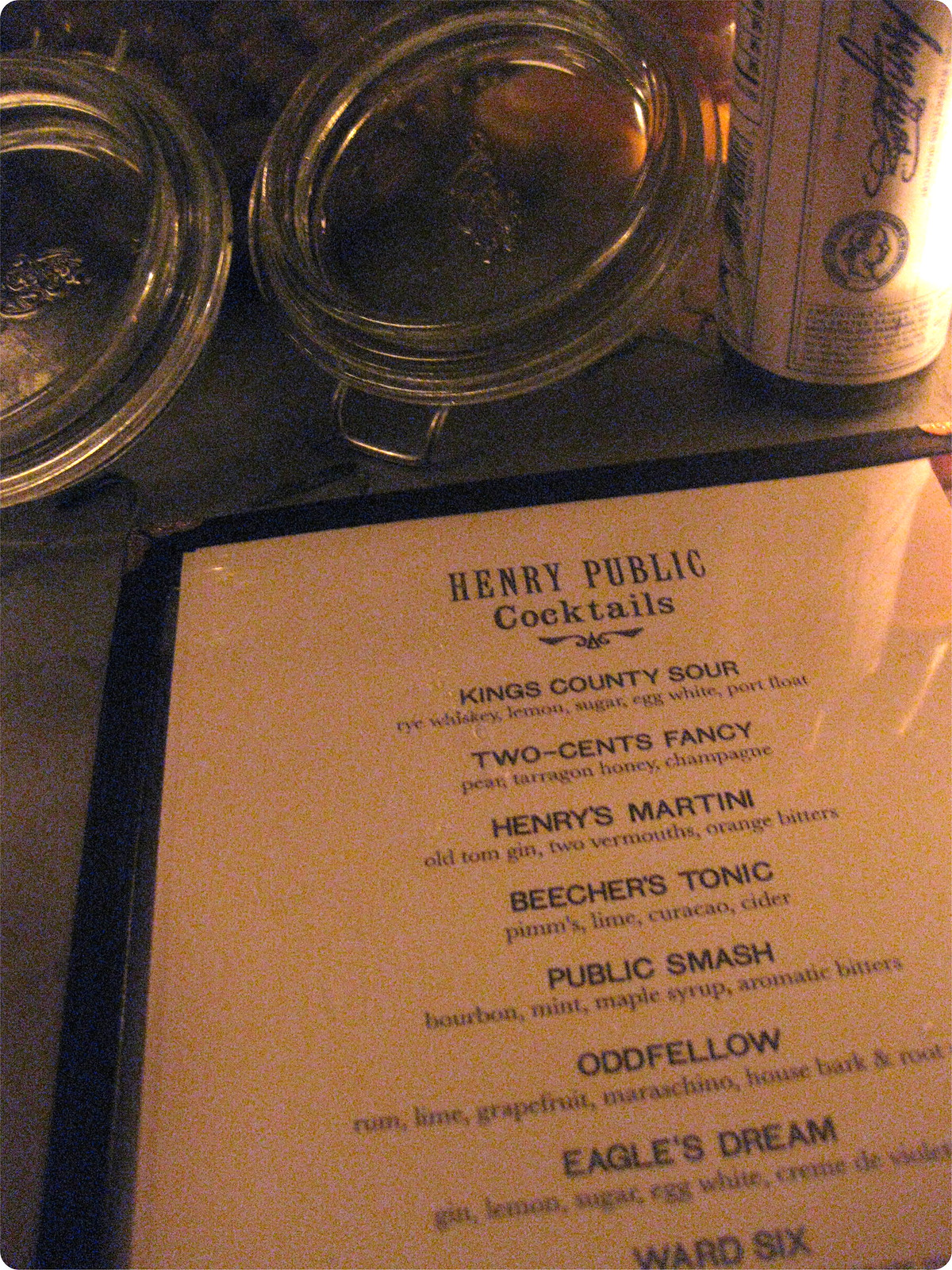This photo appears to be taken inside a pub or restaurant, focused on a detailed view of a cocktails menu on a table. The menu, bordered in black with white pages and black text, prominently reads "Henry Public Cocktails" at the top. The list features a variety of enticing drinks: Kings County Sour (Rye Whiskey, Lemon, Sugar, Egg White, Port Float), Two Cents Fancy (Pear, Tarragon, Honey, Champagne), Henry’s Martini (Old Tom Gin, Two Vermouth, Orange Bitters), Beecher’s Tonic (Pimm’s, Lime, Curaçao, Cider), Public Smash (Bourbon, Mint, Maple Syrup, Aromatic Bitters), Oddfellow (Rum, Lime, Grapefruit, Maraschino, House Bark and Root), and Eagle’s Dream (Gin, Lemon, Sugar, Egg White, Crème de Violette). The last drink listed is Ward 6, though its ingredients are not legible. At the top of the image, two glass jar lids are visible, and to the right, there is a can with blue lettering, likely an alcoholic beverage, with partially visible nutrition facts.